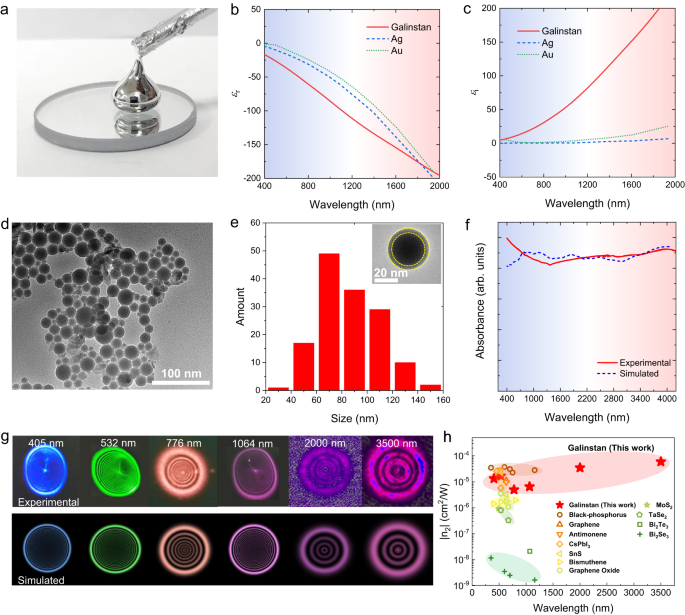The page appears to be educational material related to scientific studies, displayed on a white background and divided into eight labeled images (A-H) across three sections. The top third contains images A, B, and C; the middle third contains D, E, and F; and the bottom third contains images G and H.

Image A portrays what seems to be a drop of metal, resembling either mercury or a Hershey’s Kiss, on a mirrored surface. Image B is a graph featuring Gallenschein Aging AU, likely involving gold and silver, with a focus on wavelengths in nanometers. Image C, another wavelength chart, shows different values moving from left to right and from the bottom to the upper right.

In the middle third, Image D depicts cells or molecules as seen under a microscope. Image E is a red and white bar graph labeled "size." Image F illustrates both experimental and simulated data across a wavelength spectrum.

In the bottom third, Image G has a set of two rectangular images with black backgrounds, each displaying six colored circles (blue, green, peach, light purple, dark purple, and pinkish-purple), likely representing light readings with their corresponding measurements. Image H concludes with another wavelength chart, rounding out the scientific content displayed across the page.